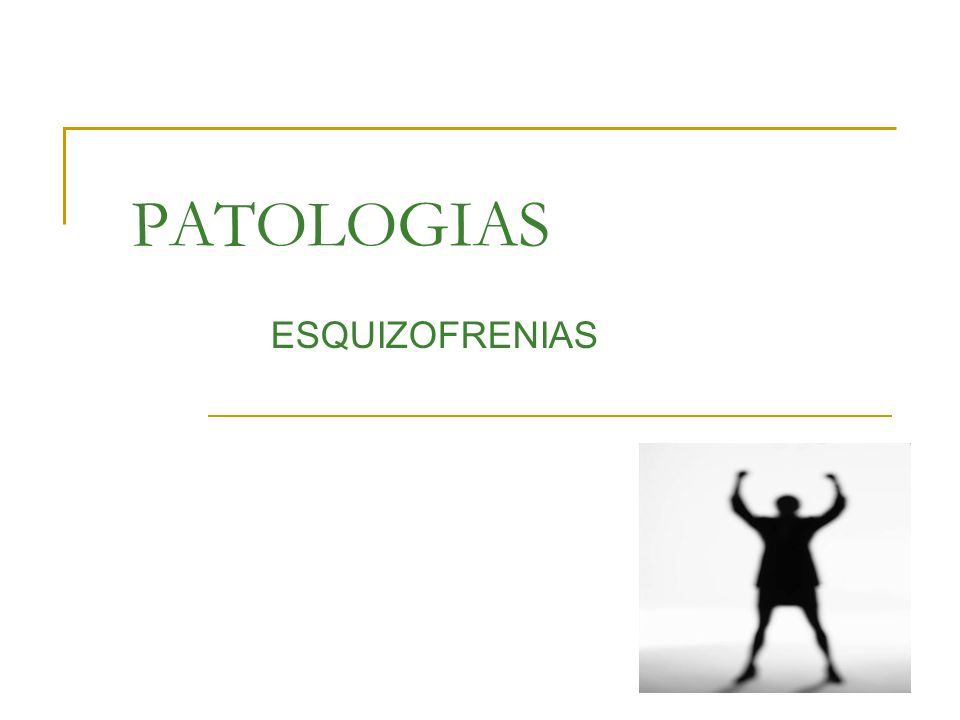In this image, set against a white background, there is a large, green, capitalized header reading "PATOLOGIAS" prominently displayed at the top left. This is followed by a subheader, also in green, which reads "ESQUIZOFRENIAS." These two text elements are separated by a thin, gold border that curves down the left side, creating an L-shape. Below the text, on the right side, there is a black and white silhouette of a figure, most likely a woman due to the skirt, with arms raised in a powerful or triumphant pose. The fists of the figure are clenched, suggesting a confident stance.